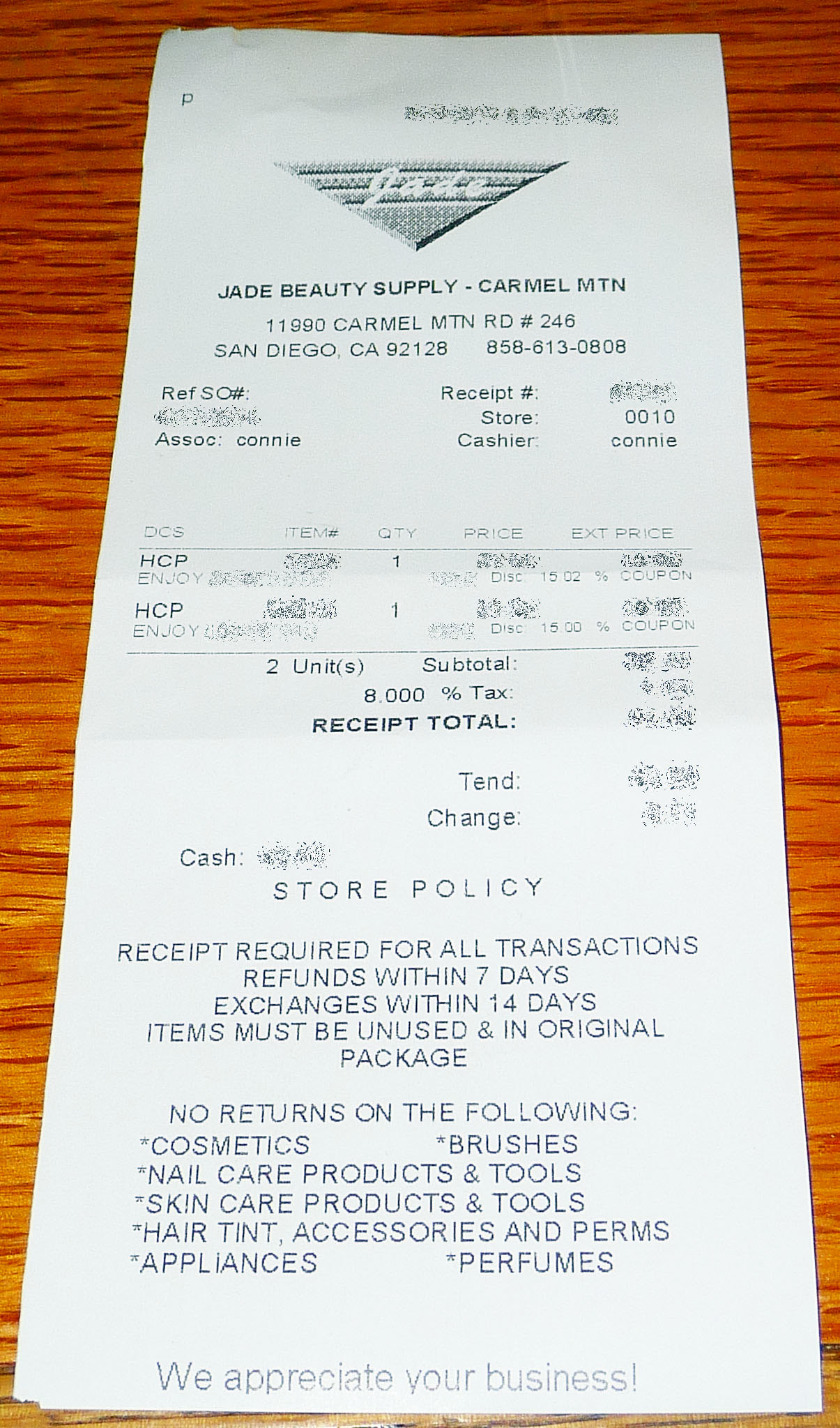The image showcases a detailed receipt from "JB Supply-Carmel MTN." At the top, there is an upside-down triangle with the initials "JB" prominently displayed in the center. The receipt details the store's address as "11980 Carmel Mountain Road, Suite 246, San Diego, California, 92128" with a contact phone number of "858-613-0808."

The receipt is from Store #0010 and was handled by Cashier Connie. It also references "HCP Client One" and notes the purchase of two units with a subtotal, plus an 8% tax.

Other receipt details include:
- Total tendered and the change given.
- Store policies such as the necessity of a receipt for all transactions.
- Refunds allowed within seven days and exchanges permitted within 14 days, provided items are unused and in their original packaging.
- A no-returns policy on specific items: cosmetics, brushes, nail care products and tools, and skincare products and tools.

The bottom of the receipt expresses gratitude for the customer's business and mentions an intent to access items for a free loan.